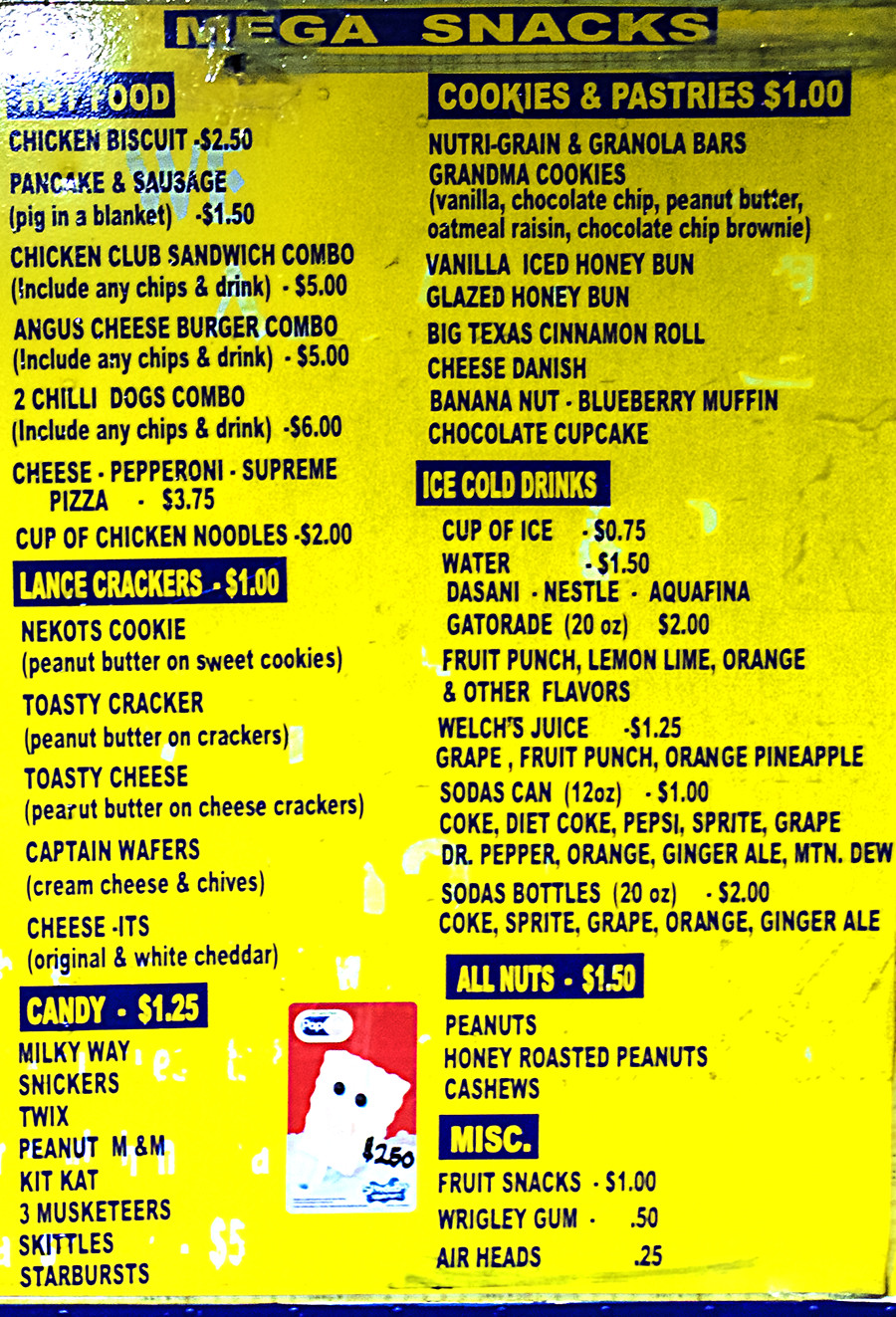The image features a menu entitled "Mega Snacks" with a hot food section prominently displayed at the top. The menu is designed with a yellow background and black text for clear readability. The main categories listed are:

- **Hot Food**
  - Chicken Biscuit - $2.50
  - Pancake and Sausage
  - Pig in a Blanket - $1.50
  - Cup of Chicken Noodles - $2.00

- **Lance Crackers - $1.00**
  - Toasty Cracker
  - Toasty Cheese
  - Captain Wafers

- **Candy - $1.25**
  - Milky Way
  - Snickers
  - Twix
  - Other assorted candies

- **Cookies and Pastries - $1.00**
  - Vanilla Iced Honey Bun
  - Glazed Honey Bun
  - Big Texas Cinnamon Roll
  - Other assorted cookies and pastries

- **Ice Cold Drinks**
  - Water
  - Welch’s Juice
  - Various Sodas

- **Double Nuts - $1.50**

- **Miscellaneous**

At the bottom of the menu is a character resembling a popsicle set against a red background, with a price tag of $2.50 next to it.